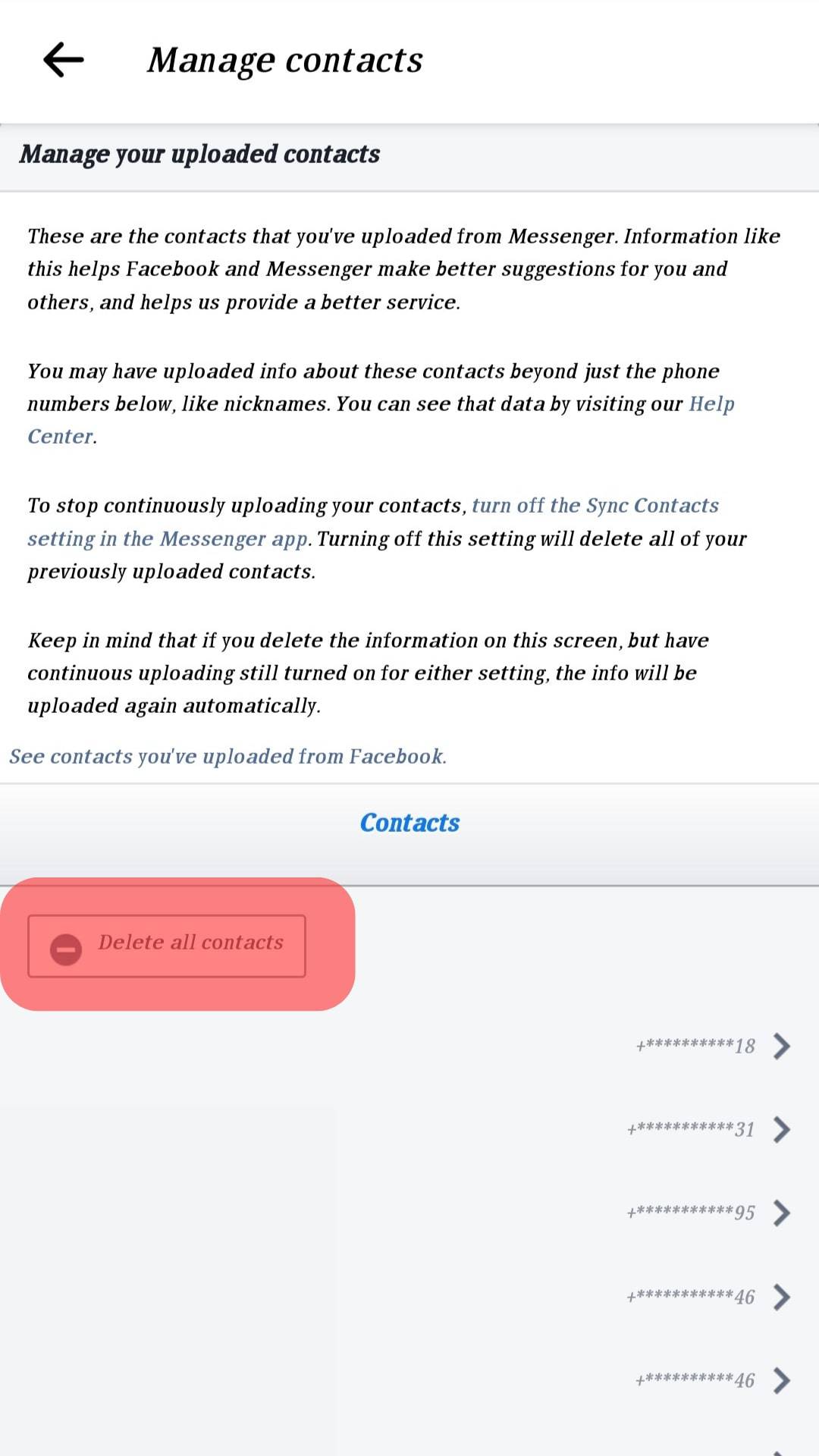The image displays a "Contacts" screen with a light gray header bar extending across the top. The word "Contacts" is prominently displayed in blue within this bar. Underneath, there is a red button labeled "Delete All Contacts," featuring a white line inside a red circle.

On the right side of the image, there is a vertical list of entries formatted as "Plus 10 Asterisks" followed by a number in blue and the word "right" in blue, repeated at different intervals. The detailed entries are:

- **+********** 18 right**
- **+********** 31 right**
- **+********** 95 right**
- **+********** 46 right**
- **+********** 46 right**

These entries are displayed in gray and blue, creating a stark contrast against the primarily white background of the page. The image's color scheme prominently features red, blue, black, gray, and white. The central area of the screen remains blank, with all the textual elements situated towards the bottom and right sides.